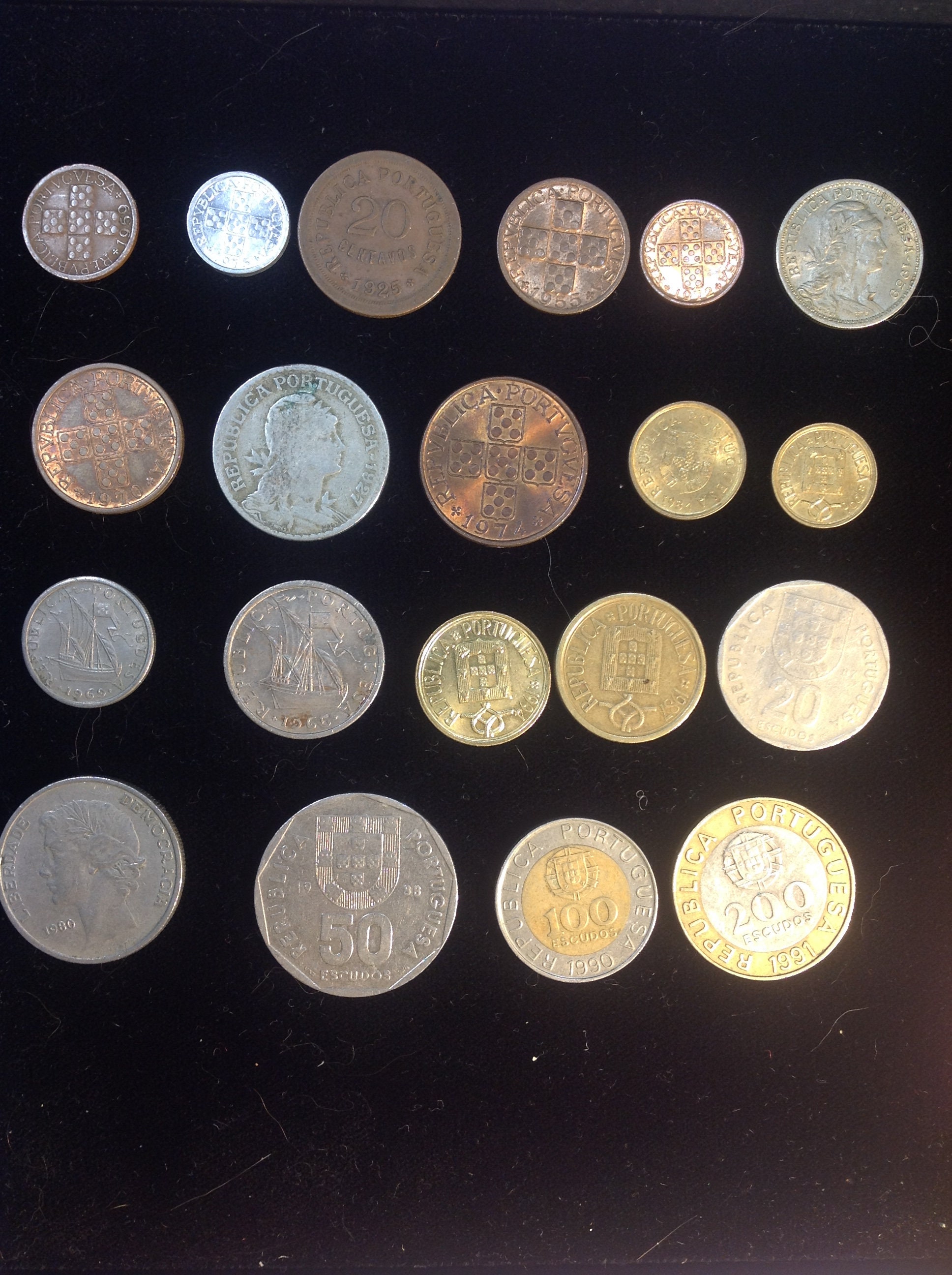This color photograph features a collection of 19 various coins meticulously arranged on a black felt background. The coins are organized in four rows: six coins in the top row, five each in the second and third rows, and four in the bottom row, creating a symmetrical and visually appealing display. The background fabric shows minute hairs and specks, adding texture to the scene.

The coins exhibit a remarkable diversity in both size and color, ranging from brilliant gold to worn pewter silver and bronze. Sizes span from coins smaller than a U.S. dime to those larger than a U.S. quarter. They include denominations such as 50, 100, and 200, though most lack numerical markings, indicating they belong to various foreign currencies or historical periods. Some of the coins show signs of rust or aging, highlighting their varied origins. Each coin features distinct designs and faces, suggesting a curated collection meant to showcase their uniqueness.